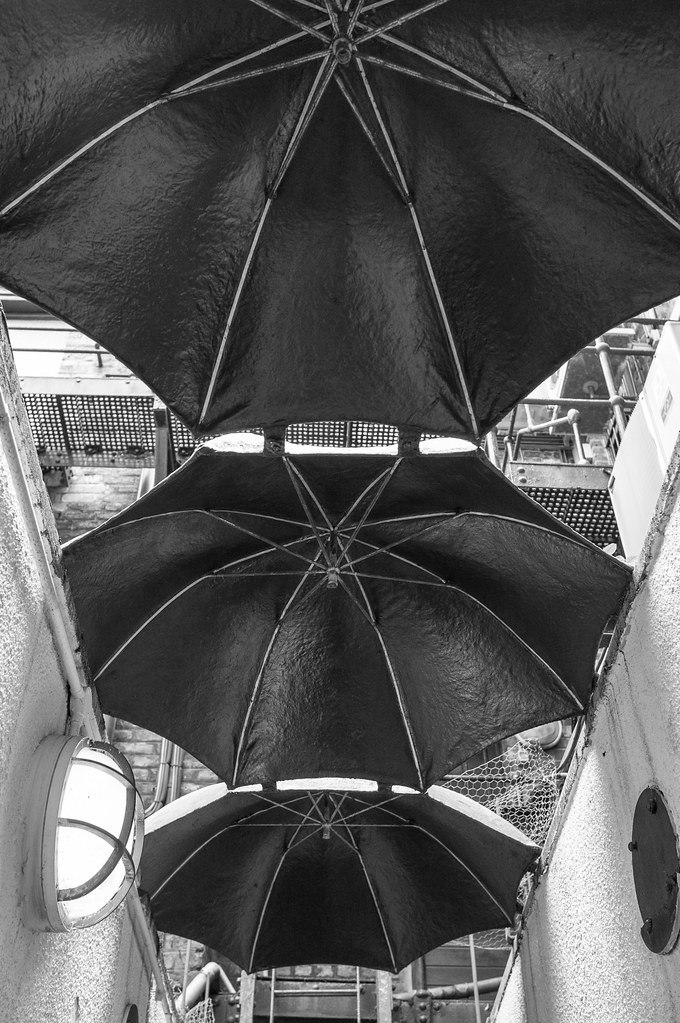This black and white photograph captures a narrow alleyway adorned with three large black umbrellas, creating a unique and artistic overhead canopy. The umbrellas, devoid of handles, appear suspended between two white concrete walls, possibly as an intentional decorative installation rather than for practical use. The largest umbrella is at the top, with each successive one slightly smaller, all featuring white or silver ribbing. The alleyway is lit by a circular light mounted on the left wall, protected by a metal cage. On the opposite wall, a similar fixture exists but seems damaged or missing. The background reveals metal railings, fences, and possibly parts of brick buildings with visible gutters, adding an industrial aesthetic to the scene. The overall impression is of an artful interplay between utility and design, transforming a simple walkway into a visually striking passage.